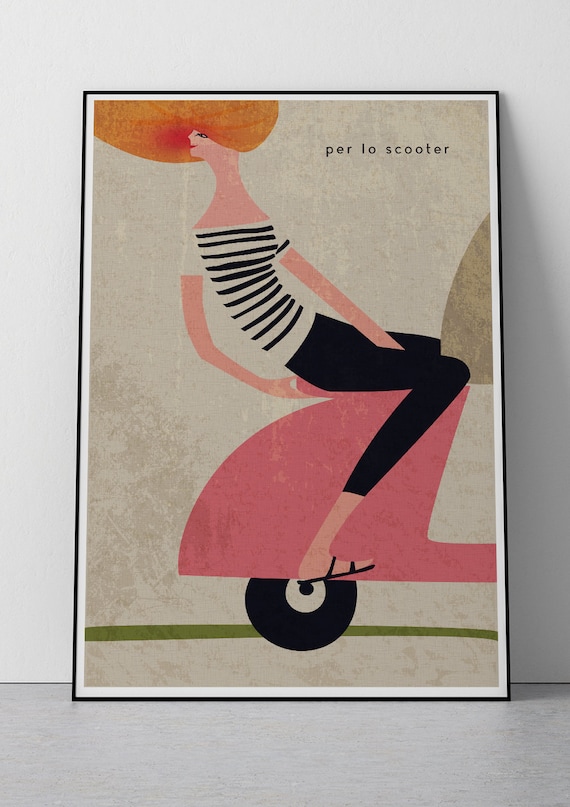The painting titled "Perlow Scooter" depicts an abstract, cartoonish image of a woman with flowing, exaggerated orange hair and thin, elongated features, riding on the back of a pink scooter. She is dressed in a white t-shirt with black stripes down the center, black stretchy pants, and black sandals. Her right hand is grasping the back of the scooter while her left hand steadies her from the middle. The woman looks precariously positioned, almost as if she's about to fall off, suggesting a sense of motion and speed. The background of the painting is a rough, canvas-like texture, and there's no discernible scenery or objects; the focus is solely on the woman and the scooter. In the top right-hand corner, the text "Perleau Scooter" is inscribed in thin black letters. This image of stylized figures against a simplistic backdrop hints at a unique and identifiable art style.